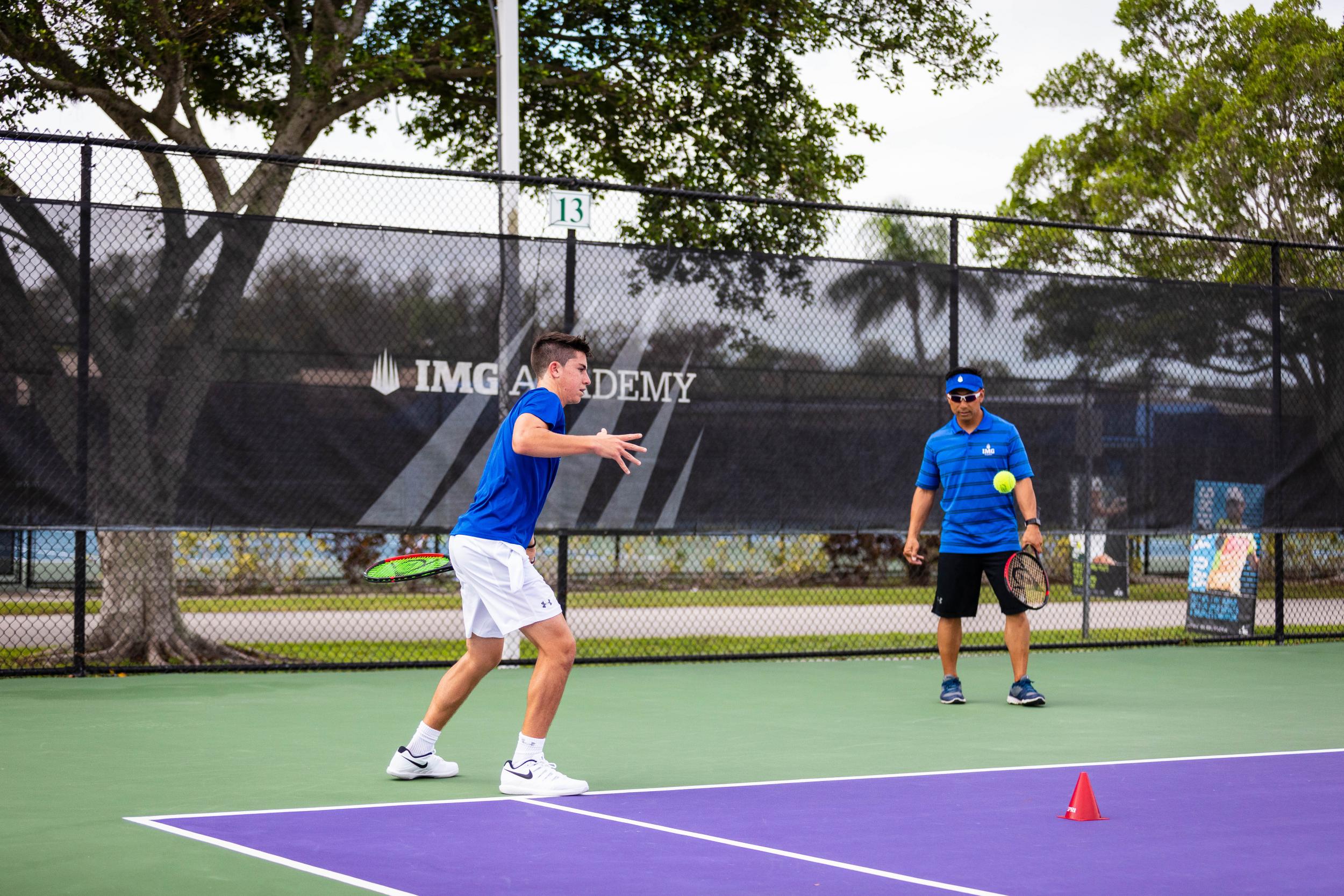In this image, two men are playing tennis on a court divided into green and purple-colored sections, with clear white boundary lines. To the left is a player in a blue shirt, white shorts, white socks, and white sneakers with a black Nike swoosh. He appears to be preparing to receive a shot, with his left arm extended and fingers outstretched. Behind him on the court is an orange pylon, likely used for tennis exercises. 

To the right is another player intently watching a tennis ball floating mid-air in front of him. He is dressed in a blue visor with a white front symbol, white sunglasses, a blue shirt with black and blue stripes and an Adidas logo, black shorts, and black and blue shoes. He is holding a tennis racket in his left hand, which is partially occluded by his body, and wears a watch on his left wrist.

The background showcases a chain-link fence with a transparent banner that reads "IMG Academy," accompanied by a wave symbol in white. Beyond the fence, there are trees and a very white, bright sky. The tennis court's vibrant colors and the players' dynamic positions suggest an active and engaging game.